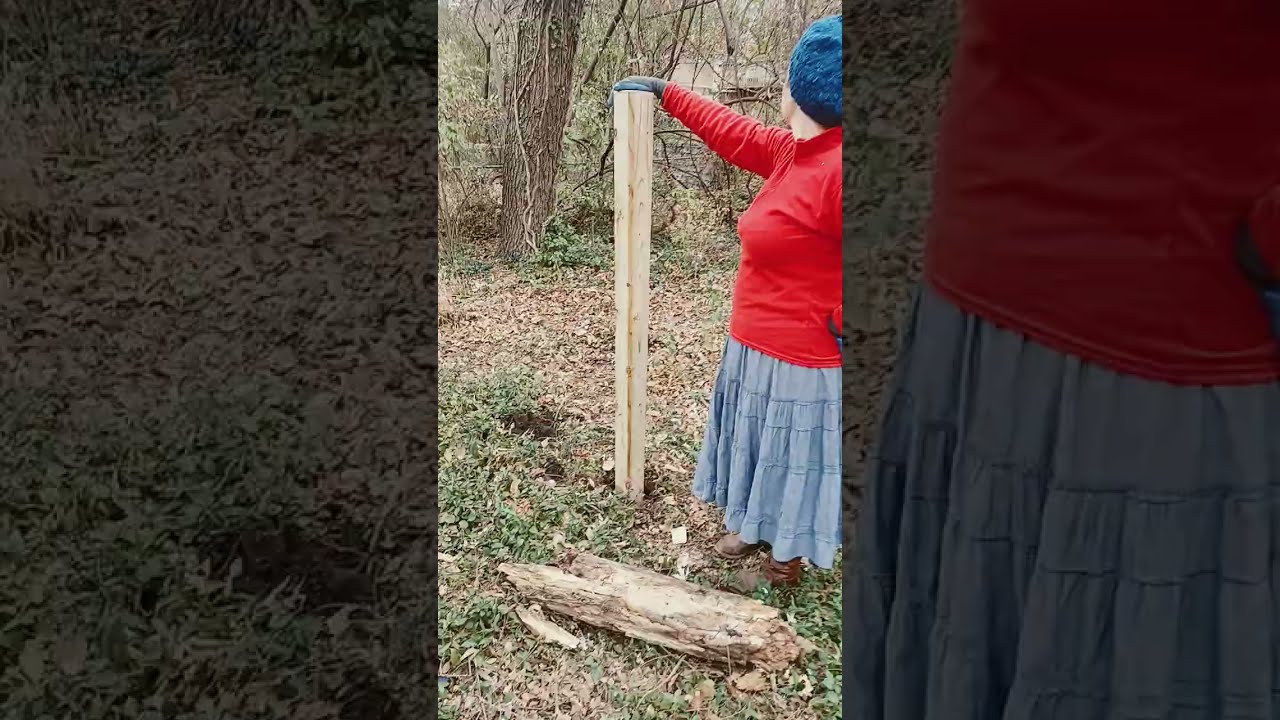This image is a color photograph in portrait orientation, embedded within a larger, darkened landscape orientation background of an enlarged portion of the same photograph. In the central photograph, a woman stands in a wooded, country-like area, characterized by green and dried grass patches and leafless trees in the background. She is dressed in a red long-sleeved sweater, a long gray or light blue skirt with frills, brown shoes, gray gloves, and a blue knitted hat. The woman faces away from the camera, looking towards the trees, with her right hand resting on a light-colored wooden post that reaches up to her chin level. A broken log lies on the ground near her feet. This photographic image, with its representational style, captures a serene and reflective moment, ideal for sharing on social media or a cell phone.